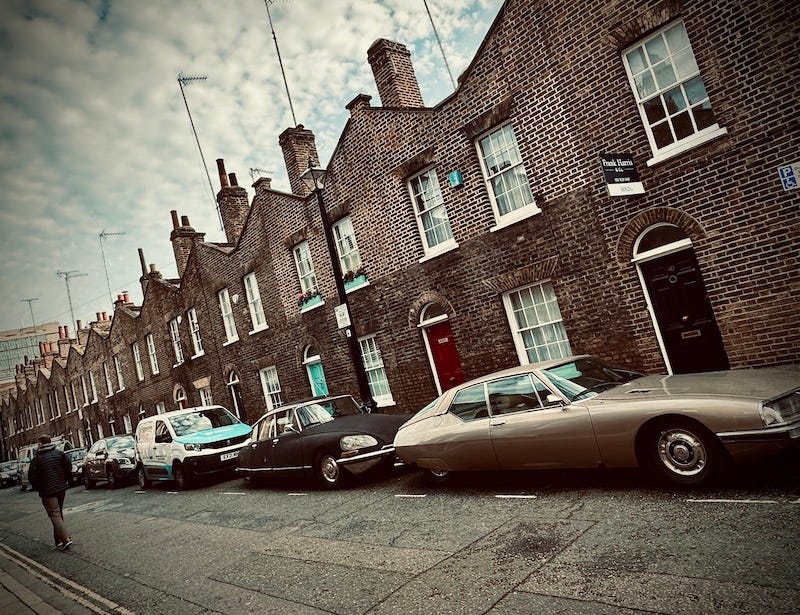In this dimly lit photo, reminiscent of an older era due to the 70s and 80s-style cars along the gray, cracked asphalt street, we see an emerald stretch of two-story townhouses. These red or brown brick buildings, uniform in design, line the street in a seemingly endless row. Each townhouse features a door with no overhang, a window adjacent, and two windows above, all with white frames and some adorned with white curtains. The buildings also boast chimneys and several metal poles, possibly antennas or satellite dishes, atop their roofs. A lone man, clad in a heavy blue coat, khaki pants, and a hoodie, walks in the opposite direction on the empty street. The parked cars, facing right, hint that the setting might be in a country where vehicles drive on the left-hand side. A sign above the first building suggests a business, with the rest appearing as homes or apartments. The cloudy sky, with patches of blue, casts a muted tone over the scene.